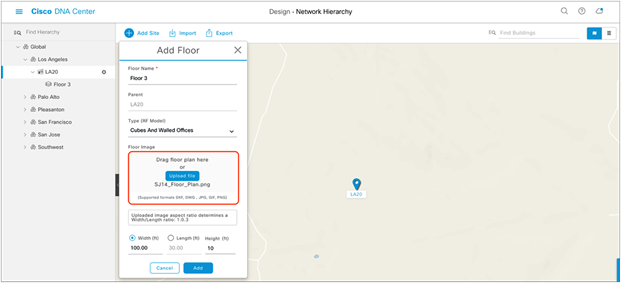This horizontal rectangular image is divided into multiple sections, each providing different pieces of information. 

At the top of the image is a horizontal rectangular banner featuring three turquoise horizontal lines with the turquoise text "Cisco DNA Center." The words "Cisco DNA" are in uppercase letters, while "Center" has only the "C" capitalized. Beneath this, in the center, is the black font text "Design," followed by the bold black text "Network Hierarchy." On the far right of this section are several icons, including a search icon.

To the left side of the image, we see a light gray background area with very small, partially legible text. At the upper left, the black text "IQ" is visible. Below this, there are several indented lines of text, which include location names such as "Los Angeles," "San Francisco," "Palo Alto," and "San Jose Southwest." Most of this text is too small to read clearly.

On the right side of the image, there is another horizontal white area with a turquoise circle containing a white X, alongside turquoise text that reads "add data." Following this are the terms "import" with an import icon, and "export" with an export icon. Below this section, there's a vertical white box. At the top of this box, in black font, it says "add floor" followed by an X. A turquoise horizontal line runs the width of this box, below which the text is difficult to decipher but appears to read "floor three." Lower down, the term "front image" can barely be made out, marked by a red rectangular oval shape surrounding it.

To the far right of this vertical box, there is an icon resembling a map teardrop pin, although no map is visible within the image. Overall, the image contains numerous elements and text descriptions adding complexity to its design.